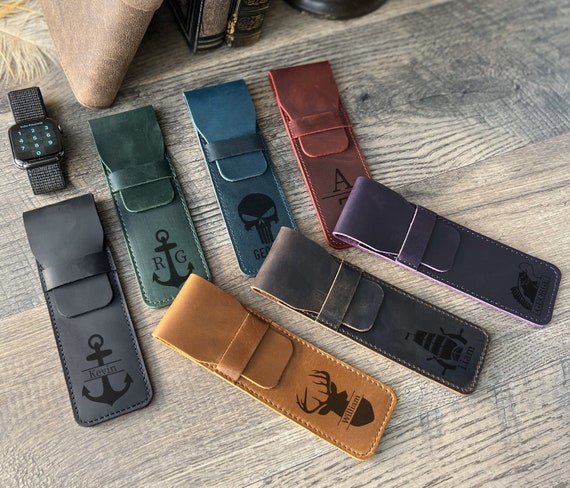This advertisement features a beautifully arranged display of seven custom-made leather cases, meticulously placed on a rough-cut shiplap board, which seems to be a table or counter. In the upper left-hand corner, a watch rests, complementing the rustic aesthetic. The cases come in various vibrant colors, including grey, green, blue, brown, lavender, burgundy, tan, and black, each exuding an artisanal charm indicative of handmade craftsmanship. 

The leather cases, potentially used for watches or other items, are adorned with personalized logos and names, showcasing their customizable nature. Visible details include an anchor with the name Kevin on a grey case, initials RG on a greenish case with an anchor, a skull on a blue case, and a deer with the name William on a brown case. Other cases have varied logos like skulls and anchors, with additional names such as Liam and some initials partially hidden.

These attractive, high-quality items hint at exclusivity and personalization, making them perfect for gifting or adding a touch of sophistication to one's personal accessories.